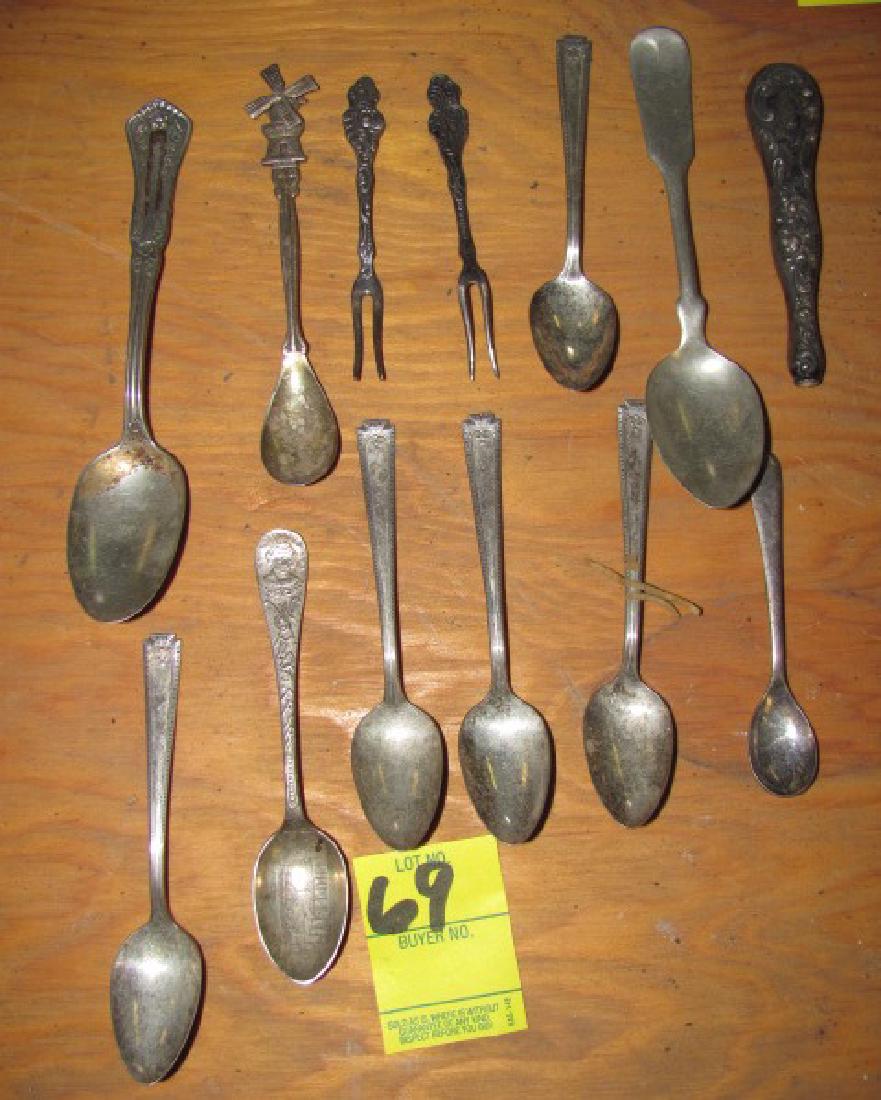The photograph captures an overhead view of a wooden table displaying an assortment of antique silverware, arranged in a neat layout. The collection consists of thirteen items: eleven spoons and two forks. Each piece varies in design, with some handles featuring ornate details such as a windmill top and others exhibiting elegant, intricate patterns. One spoon is notably incomplete, missing its bowl and displaying only the handle. The silverware exhibits signs of age, including rust, accentuating their antique and potentially valuable nature. Placed at the bottom of the image is a yellow tag labeled "Lot 69" in thick black Sharpie, indicative of an auction setting. Beneath this, the tag reads "Buyer Number," though it remains unfilled. The image is sharply focused, highlighting the vintage appeal and diverse designs of the items, suggesting a business or sales environment.